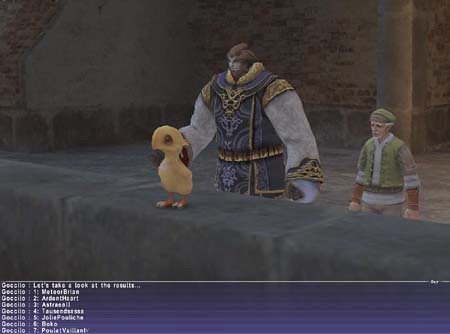The image is a still from a video game, featuring three distinct characters on a stone wall ledge with a deep green hue. At the forefront stands a yellow bird-like creature with a large beak, resembling a chick or possibly a baby dragon. Dominating the scene is a towering, giant-like man with a blue face, puffy hair, and a pointy beard, dressed in an ornate, medieval-style cloak with elaborate gold trimmings. His hands, which appear claw-like, may actually be the intricate ruffs from his heavy, brocaded sleeves. To his right stands an older, smaller man wearing a green vest, green cap, blue shirt with brown sleeves, and a belt, exuding a somewhat elephantine appearance. At the bottom of the screen, there is text that reads: "Let's take a look at the results." Behind everyone is a stone corner with a column, adding to the medieval ambiance of the scene.